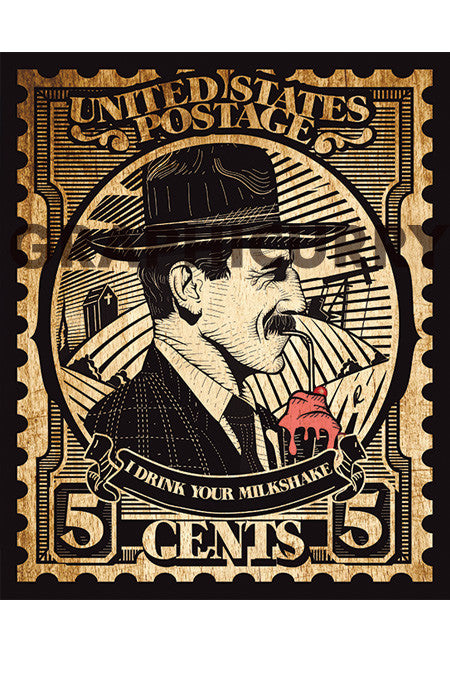This is a vintage-style cartoon illustration of a stamp, prominently featuring a black-and-white portrait of Daniel Plainview—played by Daniel Day-Lewis in the movie "There Will Be Blood." The background of the image includes a faint watermark that reads "Graphic Herpy" or a similar variation. The stamp has a cinematic ticket-shaped border with yellow accents, giving it a distinct political cartoon style.

The top of the stamp bears the text "United States Postage," and the bottom indicates its value with the number "5 cents," repeated for emphasis. In the center of the stamp, Daniel Plainview, dressed in a suit and a top hat, sips from a black glass containing a pink milkshake topped with a red cherry. Beneath him is the iconic movie quote, "I drink your milkshake."

Subtle details in the background depict a church to the left and oil rigs to the right, symbolizing key elements from the film. The overall aesthetic combines vintage postage, cinematic elements, and political cartoon illustration to create a unique and detailed piece of artwork.